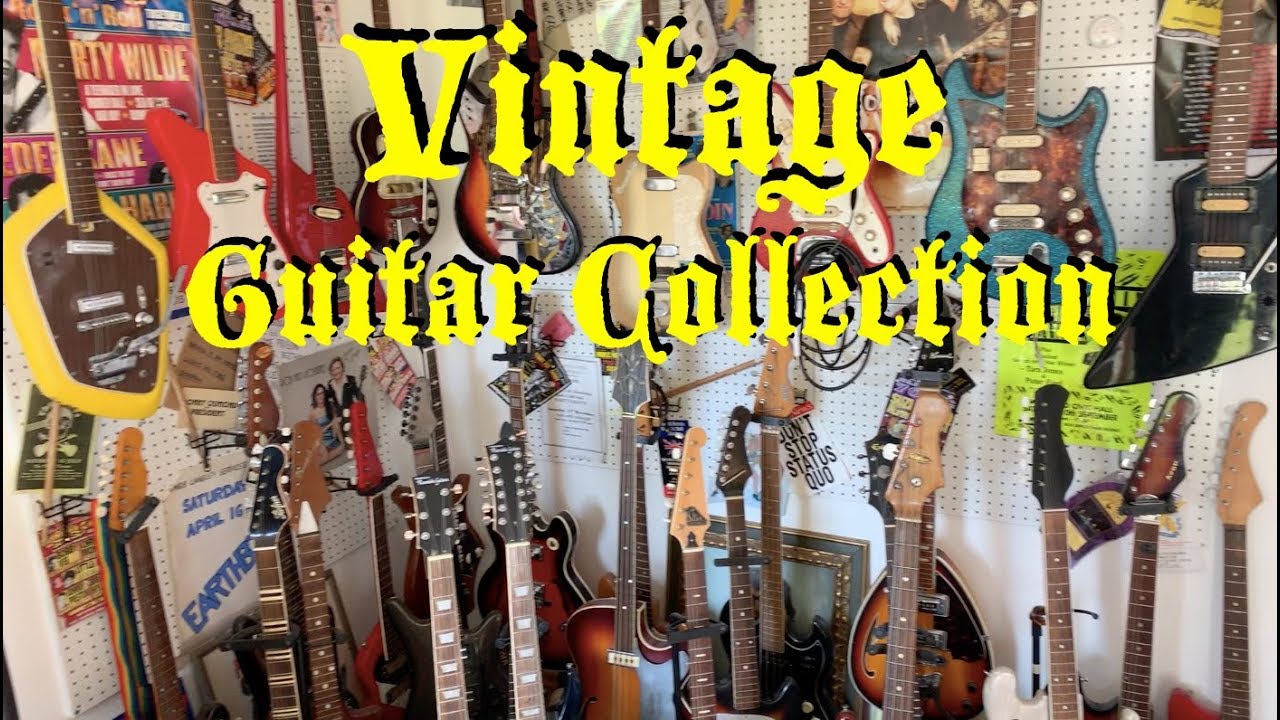This vibrant image showcases a vintage guitar collection displayed against a backdrop of white and pegboard walls. Centered at the top, in a fancy yellow font, the text "Vintage Guitar Collection" spans two lines, with "Vintage" on top and "Guitar Collection" below. The pegboard is adorned with a diverse array of over 30 guitars, predominantly electric, in various colors including yellow, red, black, orange, brown, and tan. These guitars vary in size and shape, with some hanging on the wall while others stand on the floor. Adding to the visual interest, the walls feature numerous posters and signs, including ones with messages like "Don't Stop Status Quo," and posters with red and blue backgrounds. On the left side, there's a noteworthy yellow guitar, flanked by two red ones and a black one. To the right, tan, red, blue, and black guitars are notable, with several brown guitars seen below. The collection exudes a rock-and-roll vibe, echoed by the graphic elements and the gothic typeface of the central text.